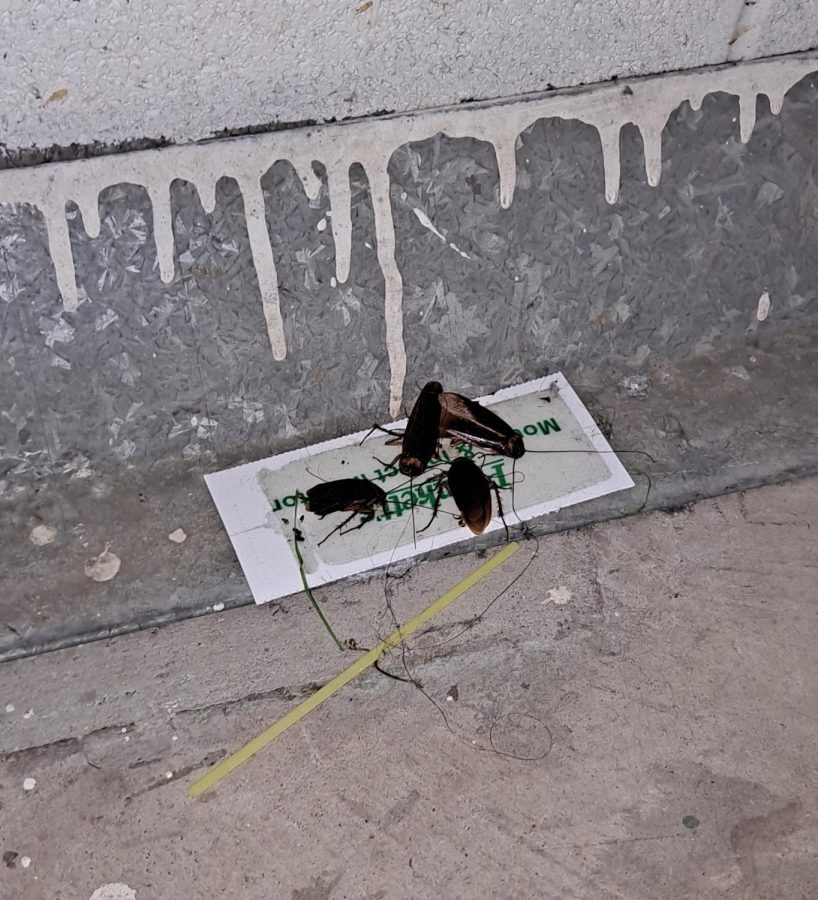The image depicts four dark brown cockroaches, each with long antennas, lying dead on a white rectangular sheet of paper, which resembles a glue trap. This trap is placed on a lighter gray cement ground, possibly in an alley or similar setting. The ground is adjacent to a gray wall, from which dry, white paint drips down toward the foundation. The wall appears to be composed of painted bricks, suggesting a chromatic contrast between the foundation and the painted surface above. Besides the roach trap, there is a distinct yellow straw on the cement ground, adding an additional element to the scene. Printed in green, some words can also be seen on the sheet of paper, although they are not clearly readable in this image.